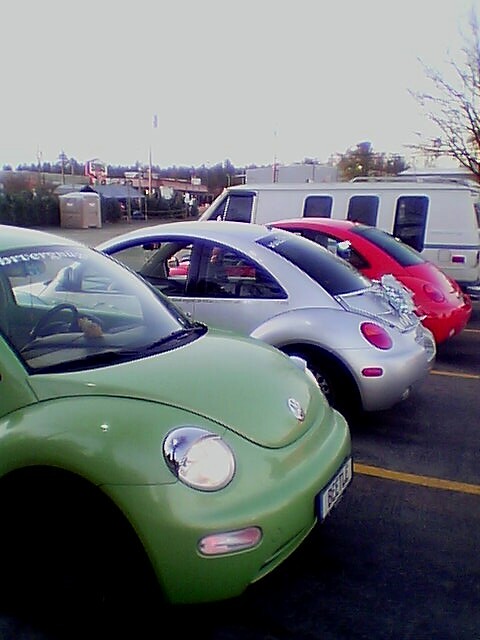The color photograph, taken in portrait orientation, depicts a parking lot with dark asphalt, which appears almost black in some areas due to shadows and image quality. Yellow lines on the tarmac differentiate the parking spaces. In the foreground, three Volkswagen Beetles are aligned diagonally: the nearest being lime green with its headlights on and facing right, followed by a silver Beetle, and furthest away, a red Beetle, both of which are parked facing the opposite direction, showing their taillights. Behind the red Beetle, a camper van is visible. In the top third of the image, an overexposed, off-white sky is present. To the left of the camper van, distant and unclear objects are discernible, including what might be a port-a-loo, a port-a-cabin, and a small structure with a pitched roof. Trees and indistinct buildings populate the far background, possibly indicating a gas station.